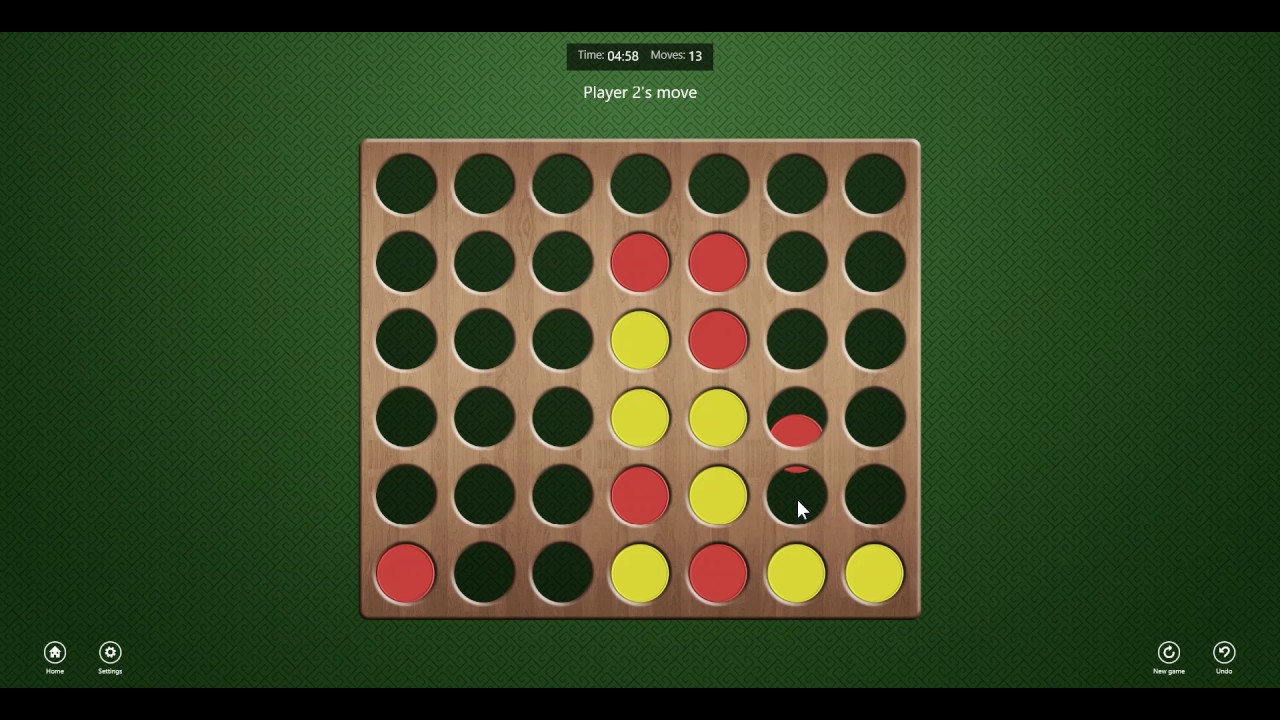This detailed caption is composed from the shared details of all three descriptions:

This image depicts a simulated board game resembling Connect 4, with the prompt indicating it is Player 2's move. In the game, players drop red or yellow discs down a vertically-oriented, light wooden grid consisting of 6 rows and 7 columns, totaling 42 circular slots. The board, featuring a neutral backdrop similar to pool table green, is shown with a red disc mid-drop. The display also notes a time of 4:58 and move number 13. Despite lacking explicit instructions and a formal name within the image, it clearly emphasizes the familiar Connect 4 gameplay mechanics, requiring players to connect four discs in a row vertically, horizontally, or diagonally. The game interface also includes small, unclear descriptions or annotations at the bottom.